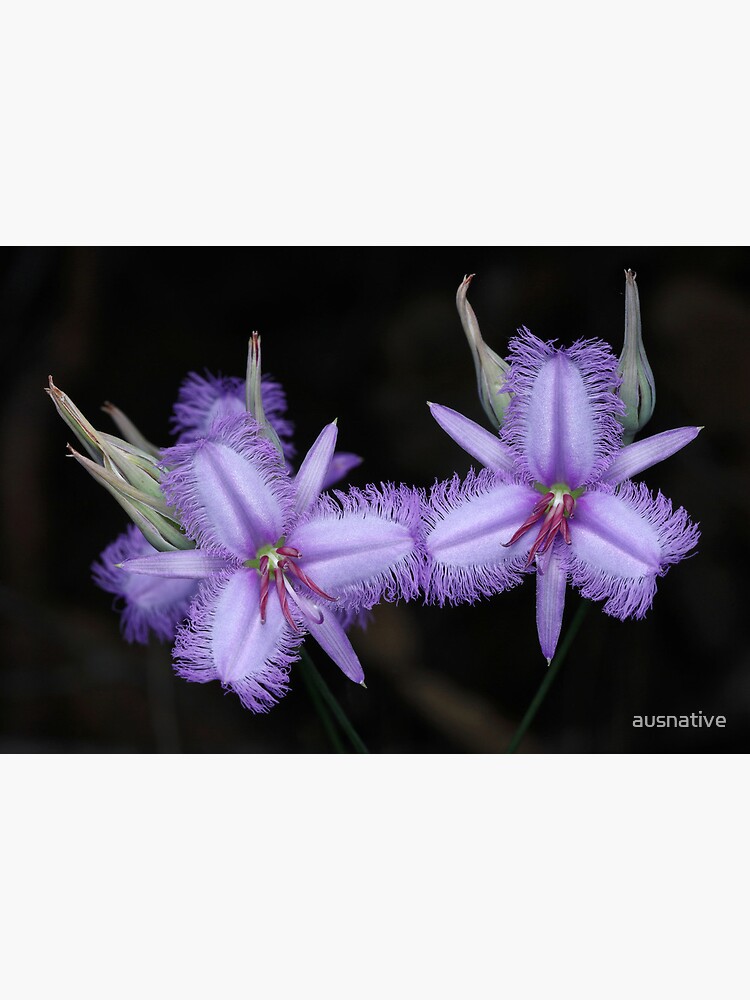The image features a striking macro shot of two unique, fuzzy purple flowers with dark purplish stems, set against a dramatic black background. Each flower’s petals are arranged in a tri-formation, with three main, thick purple petals that boast fringed, hair-like edges and sit atop thinner, pointier petals without fringes. Among the petals, delicate fine purple strands resemble hair. Interspersed with the flowers are additional green leaves and bulbous structures, creating a complex, layered look. These green elements extend from behind the flowers and contribute to their exotic appearance. Towards the bottom right is a white watermark in block font that reads "AUS Native," indicating that these flowers may be native to Australia. The combination of the dark backdrop and the vibrant, intricate details of the flowers makes them the focal point of this captivating image.